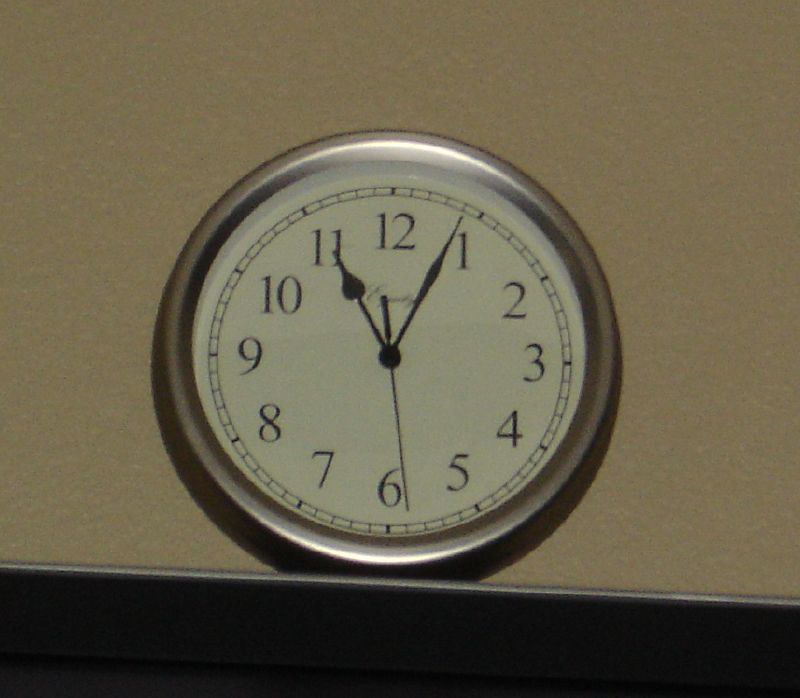This photograph captures a silver-outlined wall clock with a white face, mounted on a very beige wall above a black outcropping. The clock displays 11:04, with the second hand nearing the 30-second mark. The clock is characteristically an analog type, featuring black numerals ranging from 1 to 12, marked within a circular border with tick lines for seconds. The three hands - the hour, minute, and second - are all black, with the hour hand being shorter and bulbous at the tip, the minute hand slightly thicker with a pointed tip, and the second hand being a thin stick. The clock is positioned as if resting on or closely situated above the black structure below, with subtle reflections visible on its glass cover.